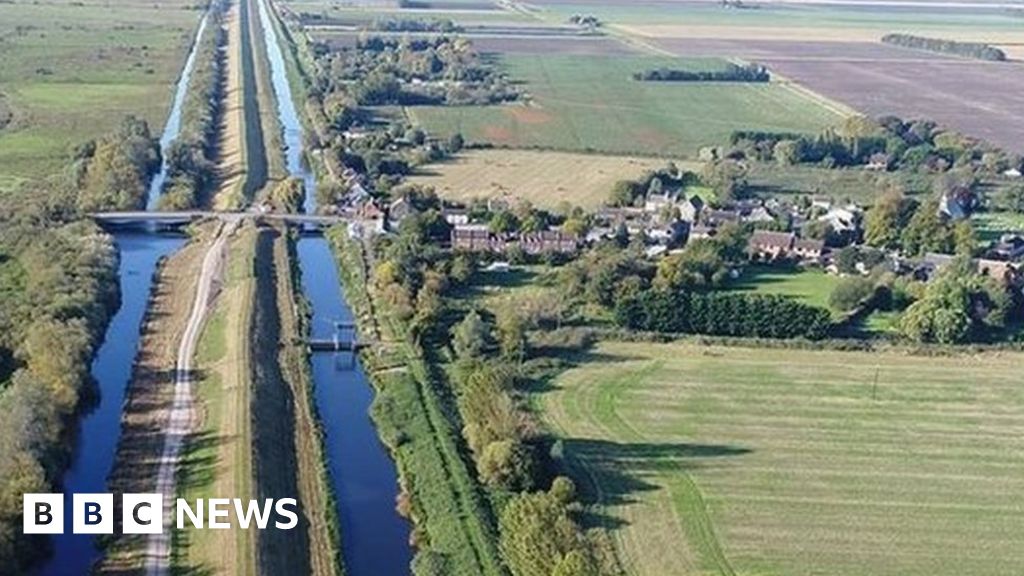The aerial photograph from BBC News features a two-level canal system with central water pathways flanked by green grass strips. A grey bridge spans the canals, connecting to a village on the right side, characterized by brown and white structures. Surrounding this settlement are vast agricultural fields, interspersed with clusters of trees and shrubbery. Most of the landscape is divided into geometric patches of farmland, contrasting with a more natural, uncultivated area of dense greenery on the far left. The scene is rich with vibrant greens and browns, illustrating the juxtaposition of cultivated land and developed village against the backdrop of winding blue waterways.